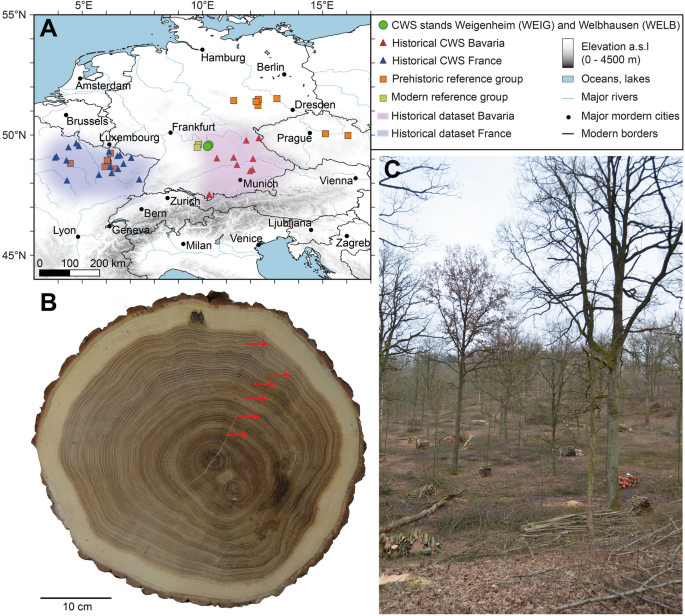The image is a digital screenshot of a detailed map of Europe, predominantly showcasing regions of France and Germany. The map includes major cities such as Amsterdam, Brussels, Luxembourg, Frankfurt, Hamburg, Berlin, Dresden, Prague, Vienna, Munich, Zurich, Bern, Lyon, and Venice. Longitude lines marked at 5, 10, and 15 degrees east, and latitude lines at 45 and 50 degrees north, frame the map. Blue represents water bodies, while modern borders are indicated with blue dashes. 

To the left, various colored shapes and text blocks serve as a key: a green circle for CWS Weigenheim (WEIG) and Welbhausen (WELB), a red triangle for historical CWS Bavaria, a blue triangle for historical CWS France, an orange square for Prehistoric Reference Group, a gray square for Modern Reference Group, a white rectangle for Historical Dataset Bavaria, and a pale blue rectangle for Historical Dataset France. The elevation ranges from 0 to 4000 meters, annotated in a white rectangle.

Adjacent to the map, there's an image of desolate landscape with barren brown land and naked trees, contributing to an overall bleak and dreary atmosphere. The forest area has numerous trees cut down, exposing their rings. Additionally, there is a close-up of a log slice, showing its growth rings with red arrows indicating measurements. The key at the bottom left indicates these rings have a diameter of about 10 centimeters.